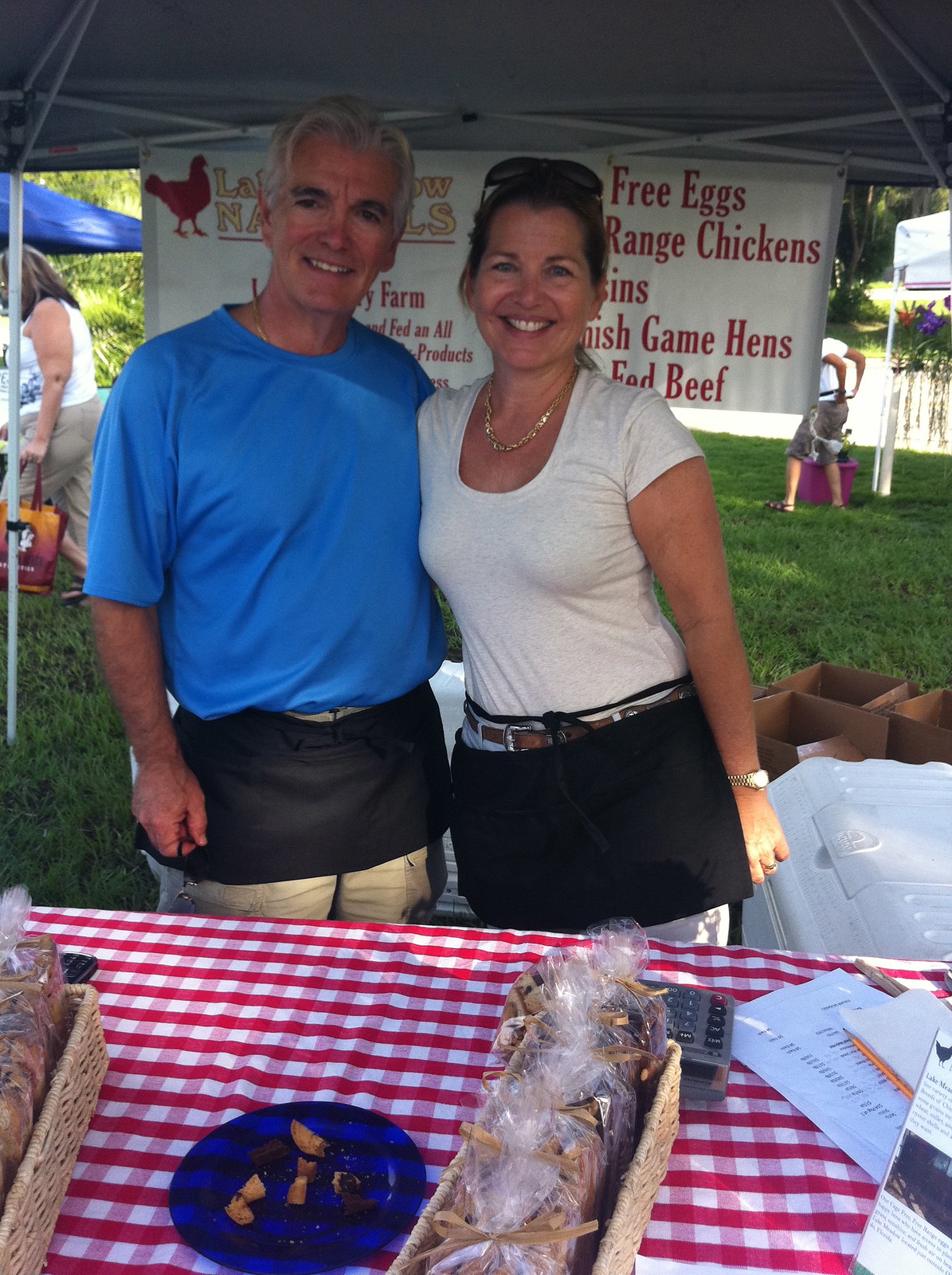This vertical rectangular photograph captures an outdoor market scene, likely at a farmer's market or a local fair, filled with vibrant and earthy tones of red, white, green, blue, and tan. At the heart of the image are a man and a woman, both smiling and seemingly posing for the camera. The man on the left sports a blue t-shirt and khaki shorts, accented by his gray hair, while the woman on the right wears a white t-shirt and white pants, with her brunette hair adorned by sunglasses perched on her head. Both are donned in aprons with pockets, hinting they might be vendors managing transactions. The table in front of them, covered by a distinctive red and white checkered tablecloth, showcases an array of items including baskets containing homemade or individually wrapped products, a blue plate with samples, a calculator, and a clipboard stacked with papers. Behind them stands a partially obscured sign listing their goods, with visible text that reads "cage-free eggs," "range chickens," "finished game hens," and "fed beef," suggesting they sell various farm products. Beyond the table, a lush patch of grass can be seen, enhancing the rural and wholesome ambiance of the scene.